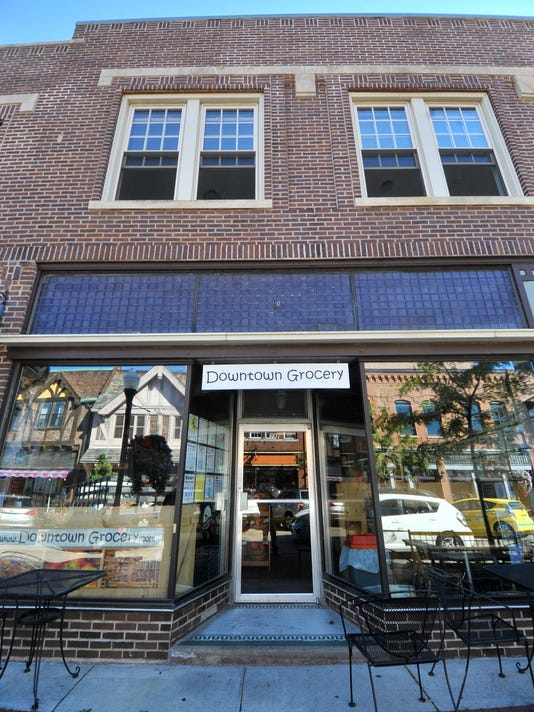The image captures a quaint two-story brick building labeled "Downtown Grocery" in playful black and white text over its front door. The storefront, which could be described as a cozy, local co-op or bistro, features large clear glass windows that reflect the bustling, traditional downtown scene around it. In front of the store, standard wire tables and chairs are set up, suggesting a space where patrons can enjoy lunch or coffee. The reflections in the windows reveal two-story homes on the left and a brick business on the right, complemented by parked cars, including a white and a yellow car. The building's well-maintained appearance, coupled with its community-centric setup, lends it a welcoming and vibrant atmosphere, typical of a lush, friendly downtown area. There are no people visible in the image, emphasizing the serene yet lively setting.